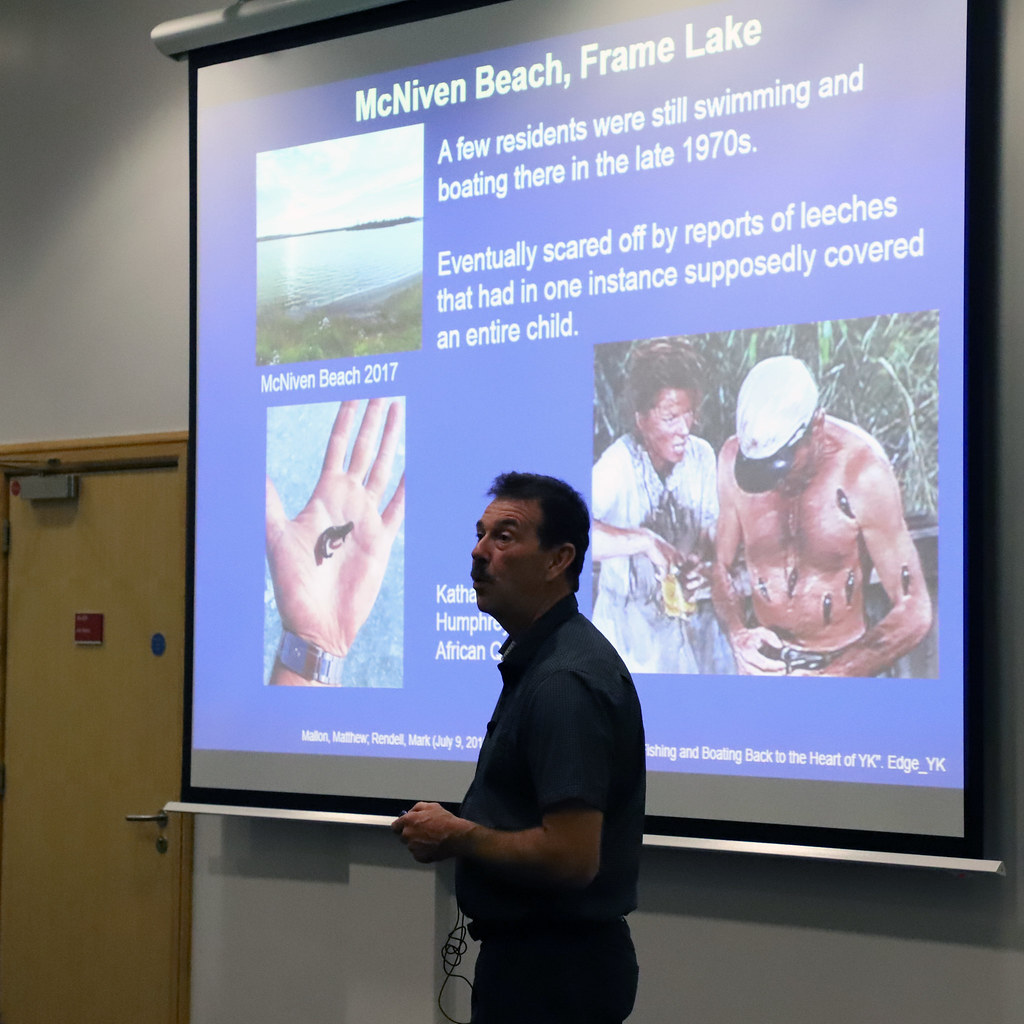A middle-aged man with short black hair and a mustache stands in front of a pull-down screen, positioned centrally in an indoor setting that resembles a classroom or conference room with tall white walls and a brown door to the left. He is dressed in a short-sleeved, dark blue or gray shirt, dark pants, and appears to have a microphone wire attached to him. The image captures him from the upper leg upwards, as he faces towards the left with his head turned slightly back. 

The screen behind him displays the title "McNiven Beach Frame Lake" at the top. To the left, there is a photo of the lake and shoreline. Below that, a hand holding a leech, with the wrist adorned with a watch, is visible. On the right side of the screen, a picture depicts a shirtless man covered in leeches, standing next to a woman, evocative of a scene from "The African Queen." Surrounding these images, there is white text detailing a story about residents swimming and boating at the beach in the late 70s, but being eventually driven off by reports of leeches, with one particular incident describing leeches covering an entire child. The background of the scene includes a gray wall behind the screen.